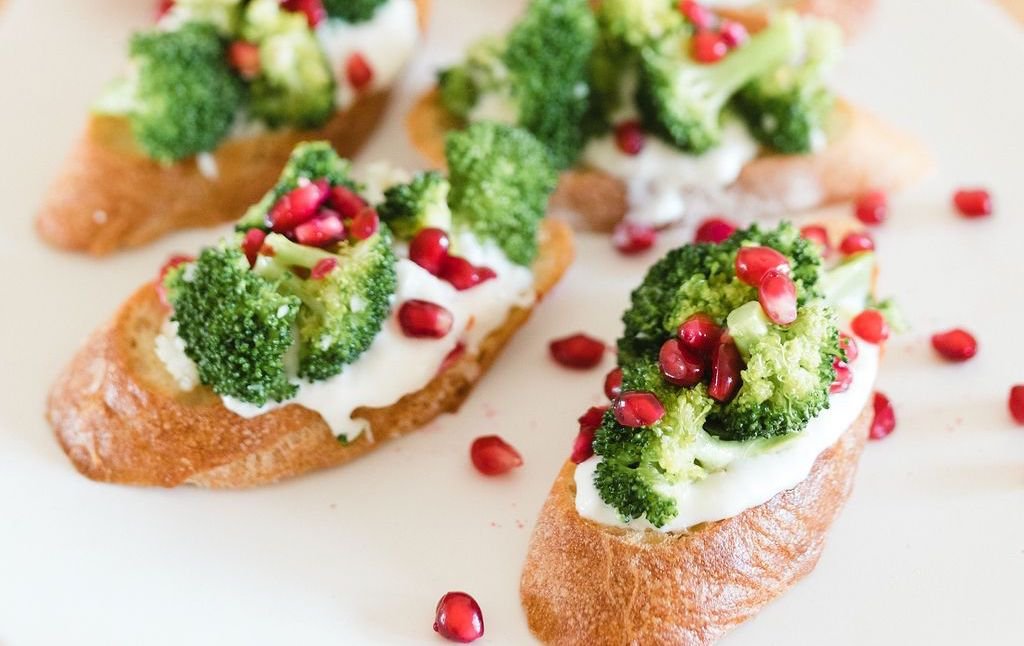The image showcases a high-quality photograph of five slices of toasted French bread with a crispy, rich golden-brown crust, displayed on a white surface. Each slice is cut at an angle and topped with a thick layer of white cream, likely cream cheese. Atop the cream are several small, green broccoli florets and deep red, oblong berries, possibly cranberries. The berries are scattered across the slices, with some falling off and lying between the bread pieces. The two slices at the bottom right are in sharp focus, while those in the upper part of the image appear blurred, adding a sense of depth to the photograph. The vibrant colors and textures suggest the dish resembles bruschetta and could easily be featured in a gourmet food magazine.